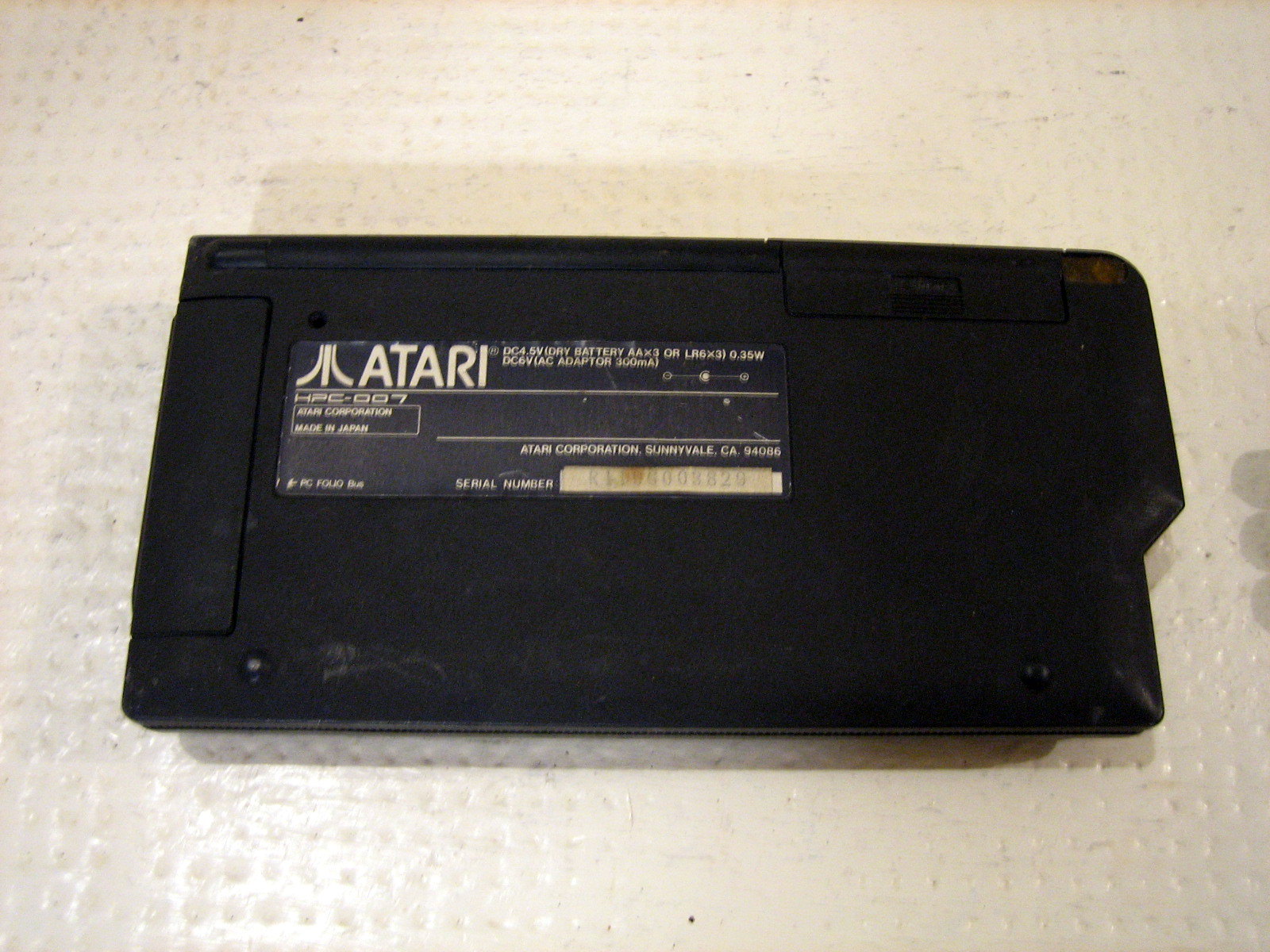The image features a black rectangular device, likely an AC adapter or battery for an Atari system, showcased against a white background. Prominently displayed on the device is a sticker that reads "A-T-A-R-I" in gold. Directly under this, in smaller text, the model number "HPC 007" is visible. Additionally, there's a label indicating "Atari Corporation, made in Japan." To the right on the sticker, one can see various technical specifications, including "DC 4.5V" or "5V dry battery AA x 3," "LR 6 x 3," "0.3W," and "DC 6V AC adapter 300mA." Another section of the sticker lists "Atari Corporation, Sunnyvale, CA 94086," along with a very faint serial number written on a cream-colored paper attached to the device. The entire setup sits on a white sheet that has small holes.